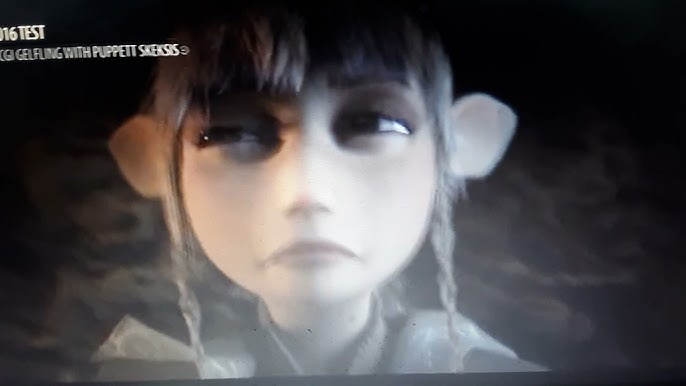This image features a computer-generated character from what seems to be a CGI film. The character is a female figure, likely an elf or magical being, with distinctive pointy ears that extend sideways rather than upright, giving her a non-human appearance. She has light brown, shoulder-length hair styled into bangs and two braids, with some strands thinly framing her ears. Her facial features are petite, including a small mouth and nose, and she possesses large, dark eyes that contribute to her almost mouse-like visage. Her expression in the image appears frowning or wary, possibly squinting. The character's complexion is Caucasian, with one ear appearing light brown and the other white. She is wearing a gray shirt, although only her neck and head are visible. The background is nearly black with an indistinct, blurred shape that might resemble mountains. In the upper left corner, partially cut-off white text reads "016 Test CGI Gelfling with Puppet Skeksis."